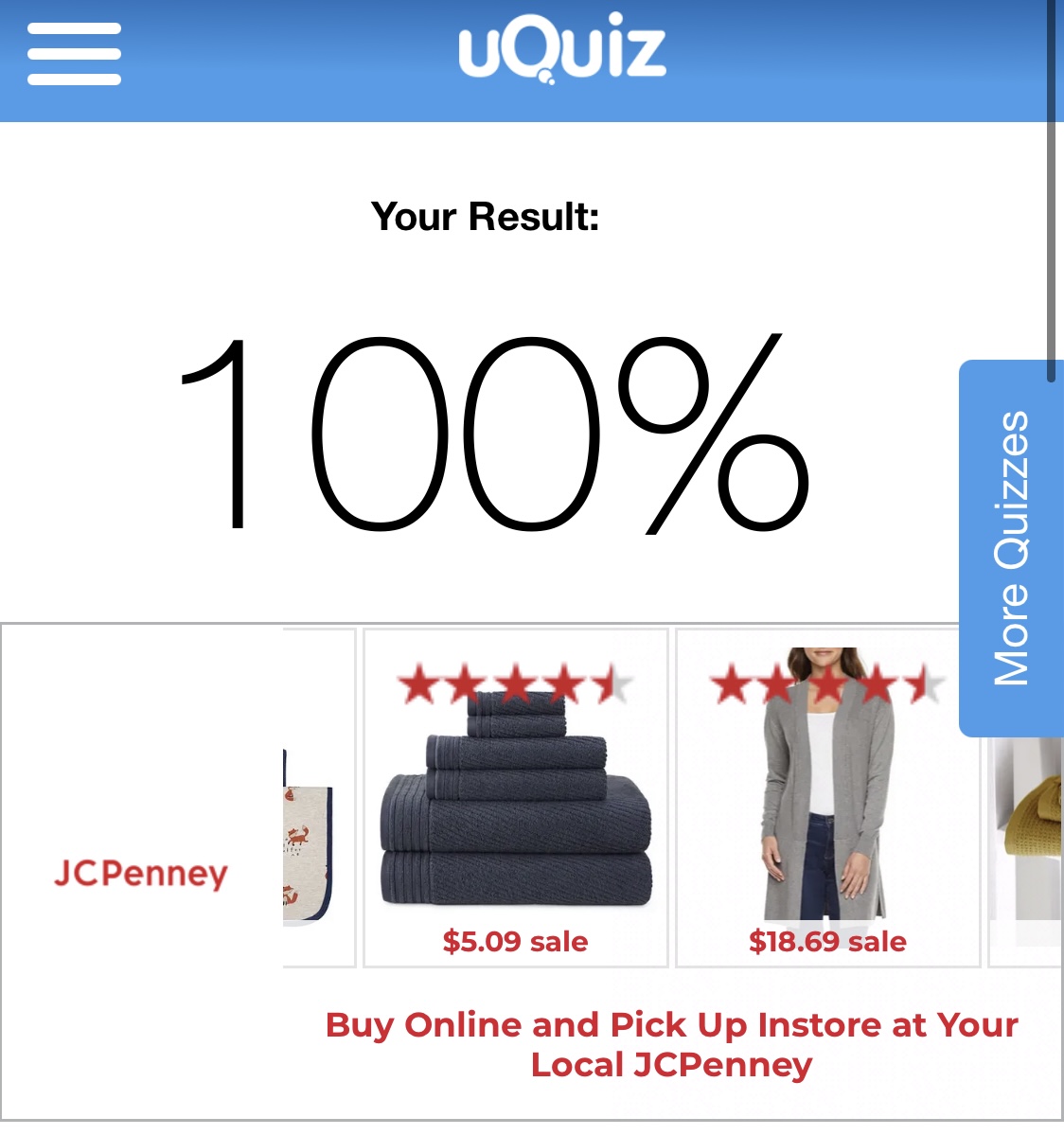The image is a screenshot displayed on a smartphone, showcasing an app or web interface named "YouQuiz," with the "Q" prominently capitalized. Central to the screenshot is a speech bubble containing the text "YouQuiz," where the tail of the letter "Q" is creatively formed by two small circles. In the top-left corner, there is a hamburger menu icon, indicating additional options.

The main content of the screenshot reveals that a user has achieved a perfect score, with the text "Your Result: 100%" prominently displayed. Below this, there are advertisements from JCPenney. The ads are presented in a scrollable format, with two options clearly visible, and partial views of adjacent options on the left and right sides, signifying the scrollability.

The first visible ad promotes bath towels, featuring two dark gray bath towels, two gray hand towels, and two gray washcloths, all priced at $5.09 on sale. This item has a rating of four and a half red stars. To the right, another ad showcases a partial view of a woman wearing a long cardigan sweater over a white t-shirt and jeans, priced at $18.69 on sale. This too has a rating of four and a half red stars. Another item, which is cut off and not fully identifiable, appears to be a tote bag. 

At the bottom of the advertisement section, in red text, it reads: "Buy online and pick up in store at your local JCPenney," accompanied by the red JCPenney logo on the left side. On the far right of the image, there is a vertically oriented tab with a light blue background and white text that says "More Quizzes," indicating additional quiz options available within the app or website.